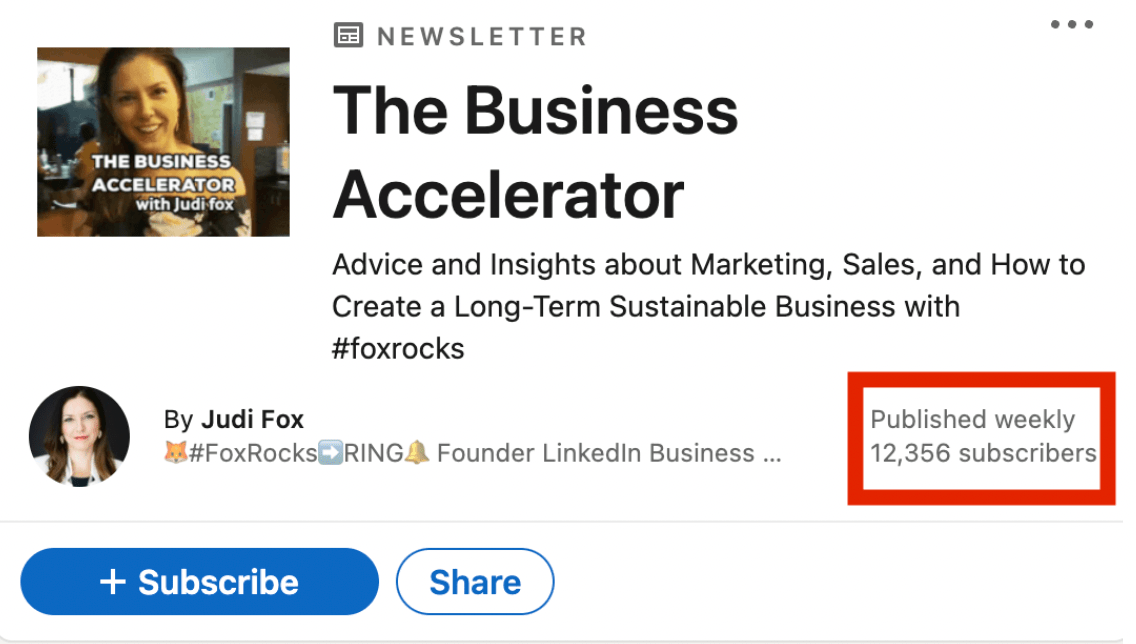Here is a cleaned-up and detailed caption for the image described:

---

The image, set against a white background, prominently features marketing content for "The Business Accelerator with Judy Fox." In the upper left-hand corner, there is a photo of a young woman, Judy Fox, standing outside an office complex, identifiable by a brown door and structural posts behind her. She is smiling brightly, has brown hair, and exudes a professional yet approachable demeanor.

To the right of her photo, the text reads "Newsletter" followed by three horizontally aligned gray dots. Below that, it states "The Business Accelerator," emphasizing that this newsletter provides valuable advice and insights about marketing, sales, and strategies for creating a sustainable long-term business, framed with the hashtag #FoxRocks.

In the bottom left corner, there is another profile image of the same woman, Judy Fox. She is depicted with long brown hair, red lipstick, and wearing a white jacket, reinforcing her consistent and professional branding. Directly next to this image, the text reads "By Judy Fox" and includes the hashtag #FoxRocks, followed by her title, "Founder, LinkedIn Business."

At the bottom right, there's a bold red rectangular box with the text "Published Weekly" inside, highlighting the newsletter's frequency and a subscriber count of 12,356. Next to this, there is a prominent blue "Subscribe" button with white font and a plus sign, followed by a white "Share" button with blue font, encouraging user engagement and sharing.

---